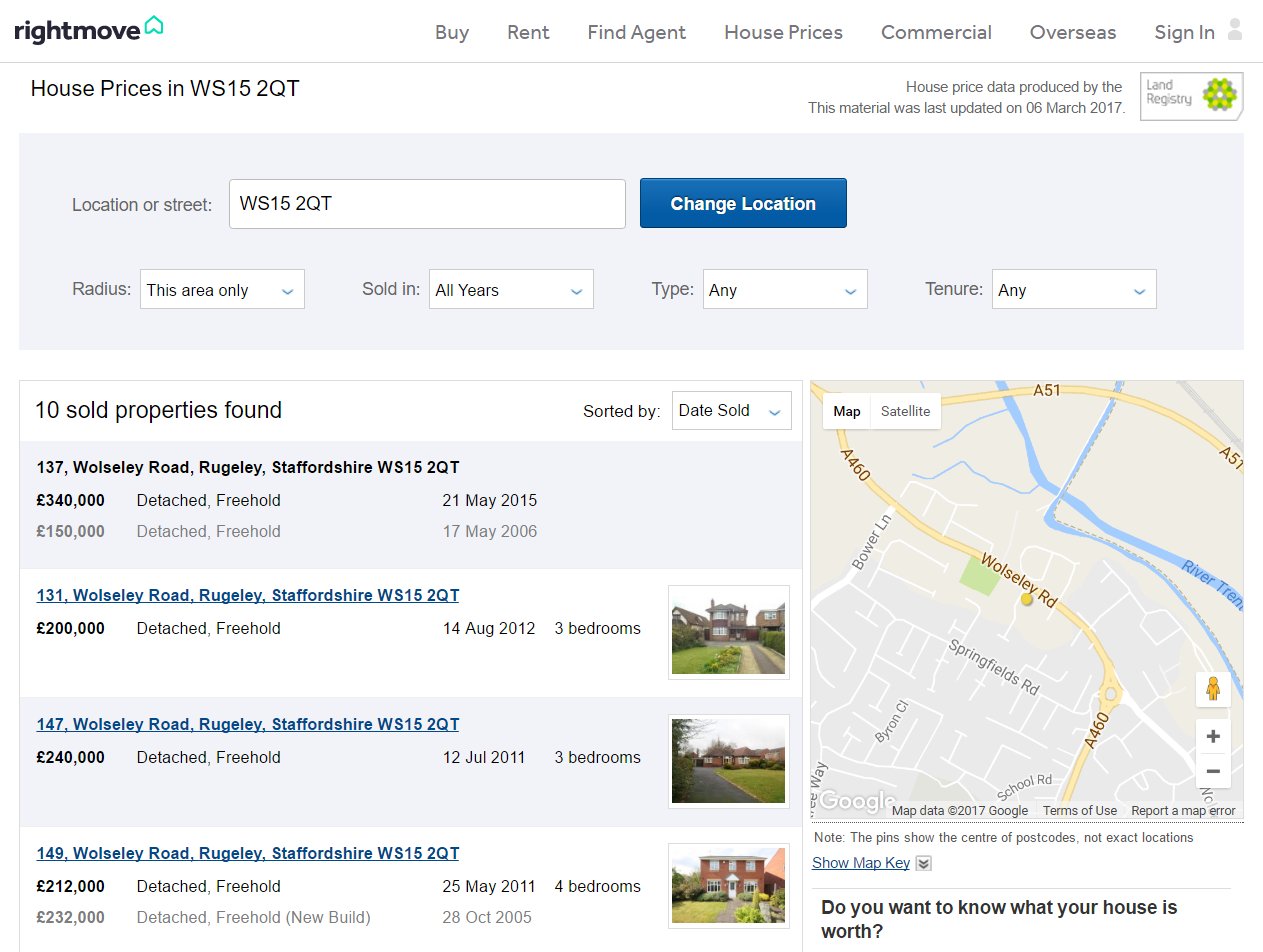A detailed web screenshot of a Rightmove webpage, showcasing property search results in Staffordshire, England. The header of the page features a variety of navigation options including 'Buy,' 'Rent,' 'Find Agent,' 'House Prices,' 'Commercial,' and 'Overseas,' along with a sign-in option for account holders. The prominent search bar displays a specific location in Staffordshire, indicating the user's interest in this area.

Just beneath the search bar, the page highlights a summary of search results, revealing that 10 properties have been found. Each property is listed with detailed information, including the sale price, type of house, and sale date. The data suggests the user is either assessing property values in the region or interested in recent real estate transactions to gauge the worth of their own house or neighboring properties.